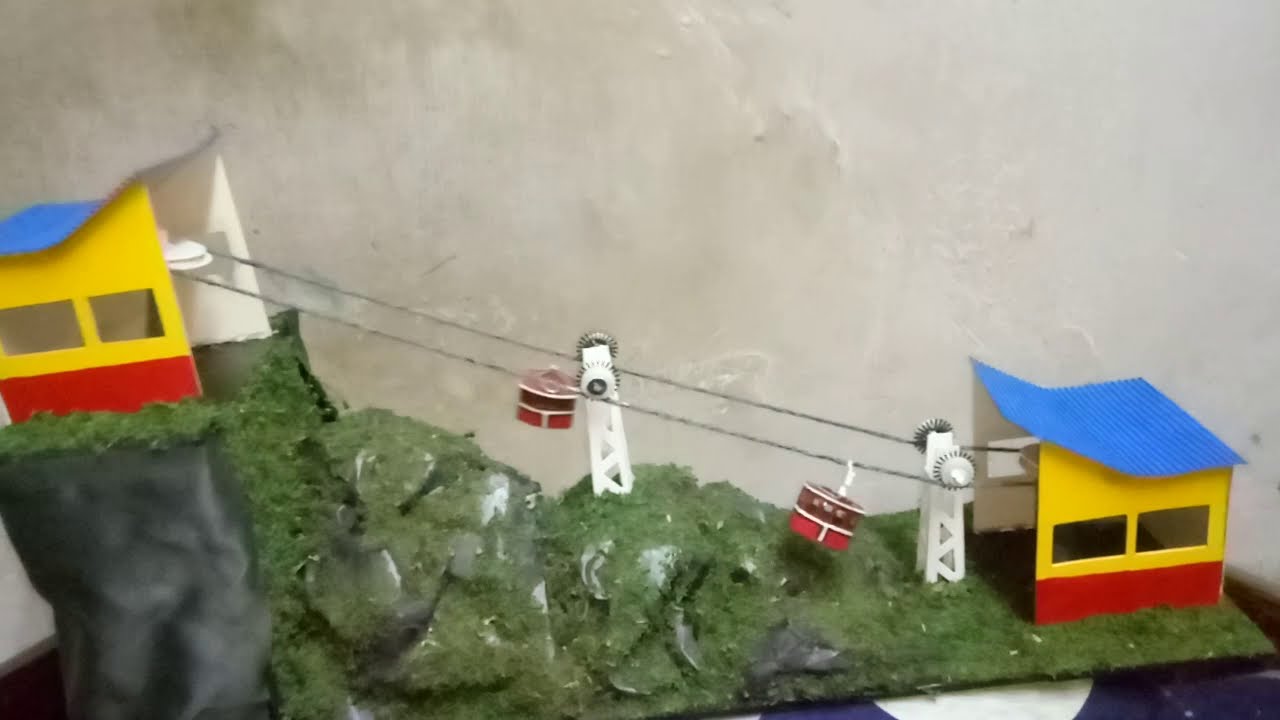This is a color photograph of a homemade model representing a funicular system on a plastic green hillside with rocky outcroppings and plastic grass. The hillside is detailed with two white towers, one positioned near the bottom and another in the center, both equipped with pulleys. Suspended from the wires are two gondolas, crafted to resemble small cabins in red, brown, and white. At the bottom right sits a building with yellow sides, a red bottom area on the wall facing us, and a distinctive blue curved roof. This building functions as a station. At the top of the hill, another similar building stands, featuring the same yellow sides with two cut-out windows, a red bottom area, and a blue curved roof that arches from the back to the front. Above this is a large, gray, mountain-like area. The wires carrying the gondolas run from the top to the bottom, with a circular area at the top where the lines are routed. The entire model is set against a plain white background, emphasizing the intricacies of the miniature funicular system.